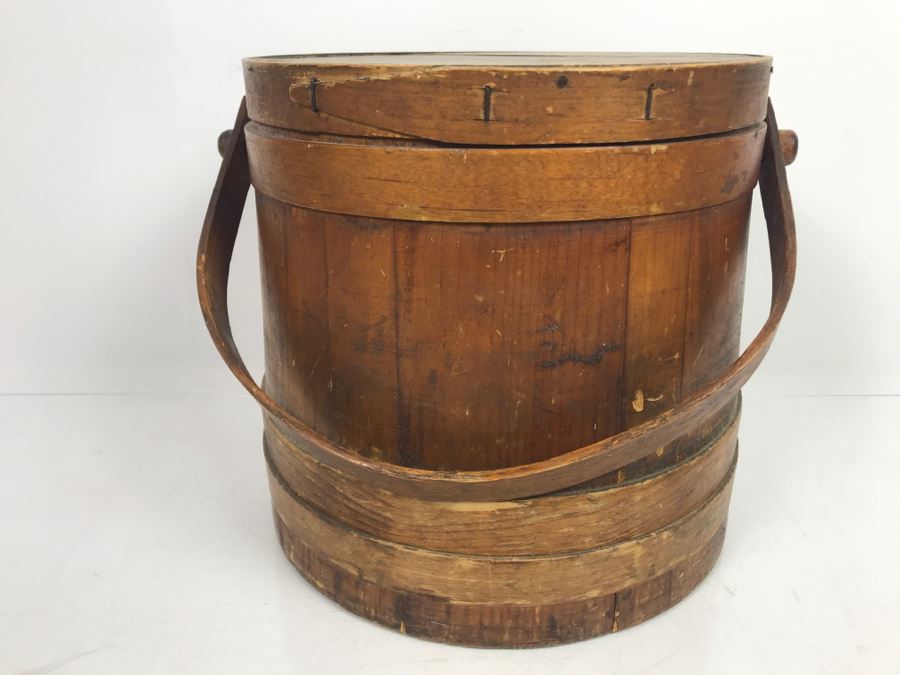The image captures a well-worn, antique cylindrical wooden bucket, centered against a white background that extends to both the wall and the hard surface it rests on. This dark brown, vintage-style bucket, likely used for storing sugar, features a distressed and aged appearance, suggesting it is a historical or antique artifact. The bucket, approximately the size of a typical five-gallon container, boasts intricate details: a wooden handle attached by two knobs to the upper rim, a lid with three vertical, darker cuts, and dual circular bands near the base and the top, each about two inches wide. The entire setup conveys an antique furniture aesthetic, with noticeable scuffs, chips, and dents adorably adding to its rustic charm.